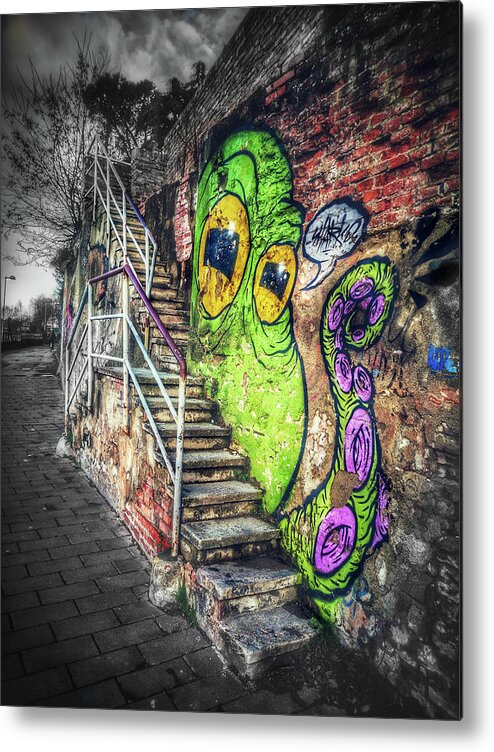This photograph captures an outdoor scene featuring an old, graffiti-covered brick wall with a staircase mounted on its left side. The image is taken from the bottom right corner, looking diagonally upward to the top left corner. The wall and surrounding area are predominantly gray, black, and rust-colored, evoking a sense of decay and age. The sky is dark and stormy, with hints of tree branches visible against it.

The staircase, which appears weathered and discolored, has a steel railing on its left side and allows for both ascent and descent, split by a landing. Further up, another staircase continues to the top of the building. The ground is paved with brick flooring, colored in dark browns and grays.

A vivid piece of graffiti art dominates the wall, depicting a large, cartoonish green octopus with irritated, oversized yellow eyes and black square pupils. One of its tentacles, adorned with purple and pink circles, stretches out to the right side of the image. The octopus seems agitated, with one eye larger than the other, and features a speech bubble scribbled in white, adding to its expressive, displeased demeanor. The overall atmosphere is one of neglected urban charm mixed with vibrant, whimsical street art.